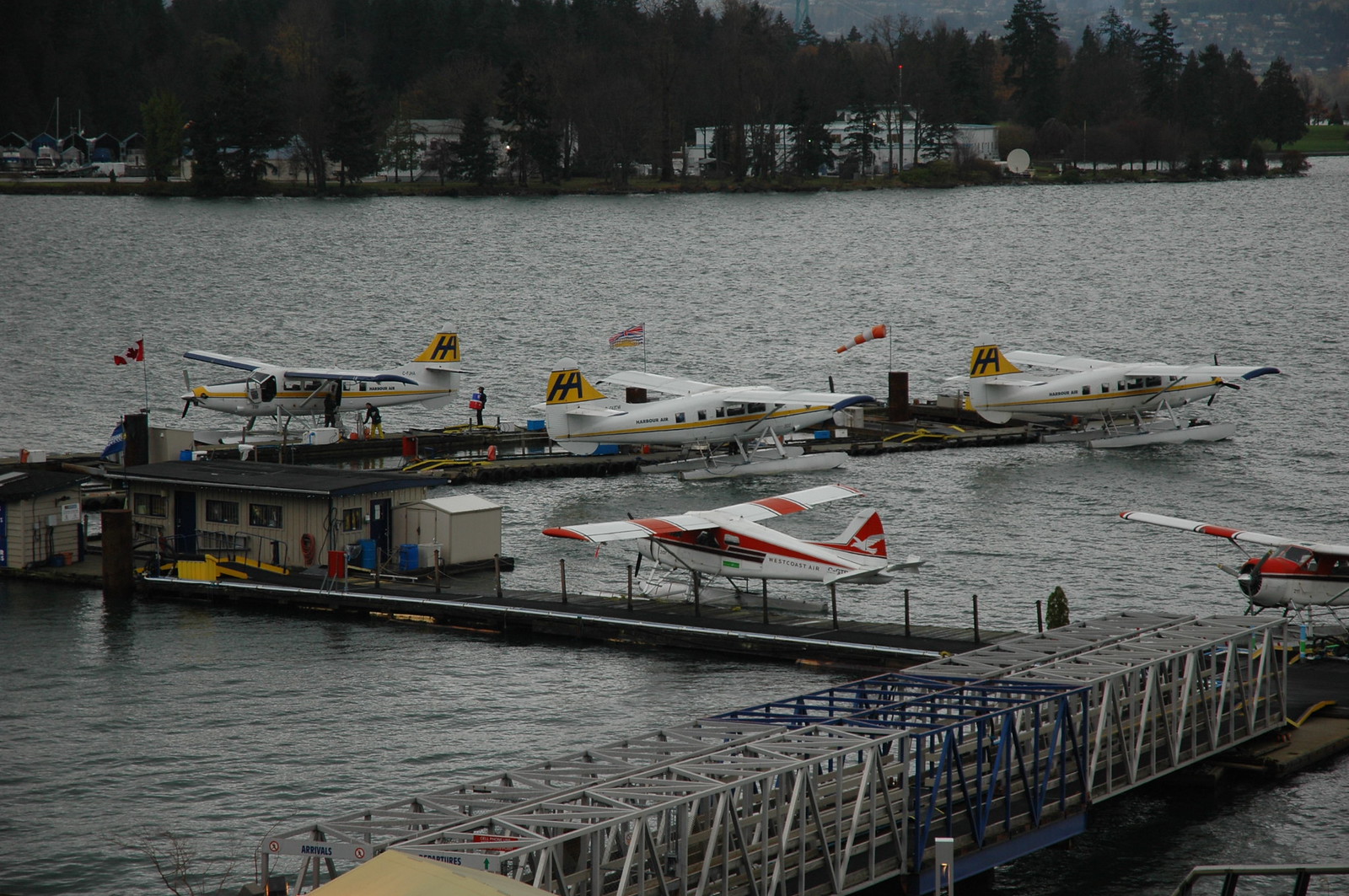The photograph captures an outdoor scene at a marina, set against a lighter blue sky scattered with darker clouds. The background reveals a dense forest with a mix of tall and shorter trees, predominantly darker green and interspersed with a line of land holding what appear to be pine or evergreen trees. Further back, a hilly landscape is visible, dotted with houses, and a body of water extends into the foreground. In this vast expanse of water, detailing five docked seaplanes is prominent. Three of these planes are uniformly white with yellow striping and yellow tags on their tails labeled "HA," while the remaining two feature red detailing. Various docks and walkways stretch out into the water, converging near a one-story building with a flat black roof, tan siding, and three visible windows on one side, plus an additional window and a door on the back. The scene is slightly dim, suggesting an overcast sky or waning sunlight.